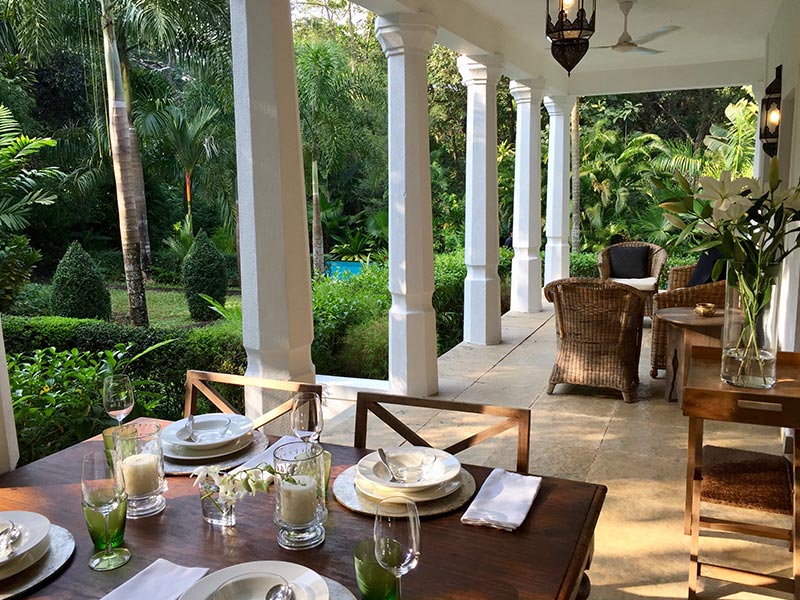The photograph depicts a grand, mansion-like residence characterized by its large white pillars and expansive porch area. Central to the image is an intricately set dark wood dining table on the porch, complete with plates, silverware, wine glasses, green-tinted drink glasses, and candles, creating an inviting dining scene. The porch itself is supported by white pillars and has a light brown flooring. 

In the background, there is additional seating featuring woven straw chairs with black cushions, as well as a decorative wooden cart table that holds potted plants with green foliage and white petals. Surrounding the porch is a lush, tropical environment with vibrant green shrubbery, trees, and palm leaves. In the distance, a turquoise blue body of water can be seen, adding to the tropical ambiance. The overall style hints at a Spanish-inspired design, enhancing the feeling of luxurious, outdoor living.